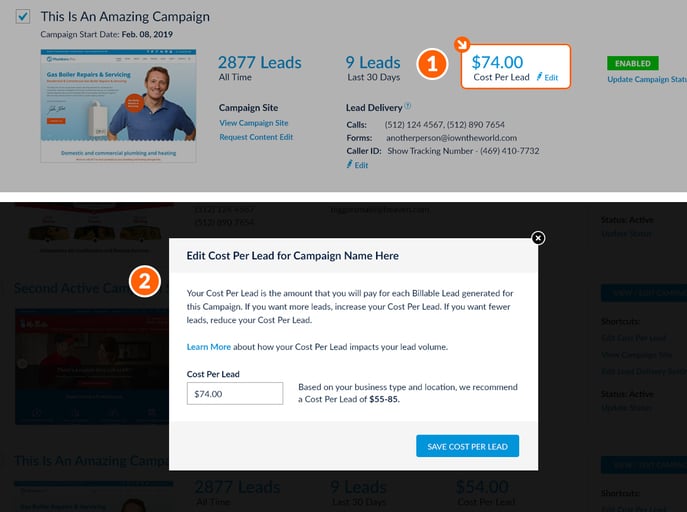The advertisement page prominently features a header that reads, "This is an Amazing Ad - Amazing Campaign Starts February 8th, 2019." It showcases a website where a smiling person stands, accompanied by some boilerplate text. To the side, it lists statistics: "2,877 leads all time" and "9 leads in the last 30 days." A marker highlights an area labeled "$74 cost per lead."

Below, the campaign's methods of lead delivery are detailed: "calls, forms, caller ID," while some text remains obscured under a dark overlay. Additionally, there is a white pop-up screen with an orange circle labeled "2." The pop-up explains, "Edit Cost Per Lead for Campaign Name Here," followed by a detailed description: "Cost per lead is the amount you’ll pay for each billable lead generated for this campaign. If you want more leads, increase your cost per lead. If you want fewer leads, reduce your cost per lead. Learn more about how your cost per lead impacts your lead volume."

The current cost per lead is noted as $74. The recommended range, based on the type of business and location, is $55 to $85. A blue button allows you to save the cost per lead, and a white X in a black circle at the upper right corner lets you close the pop-up.